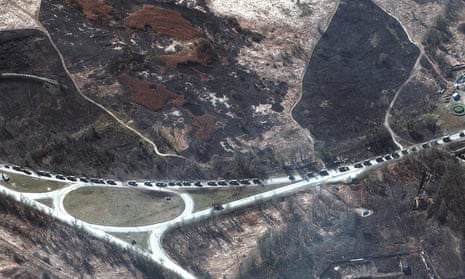This aerial photograph portrays an expansive, sparsely vegetated landscape, emphasizing a highway interchange at its center. The scene is viewed from a high vantage point, possibly from an airplane, showcasing a network of roads amidst a predominantly brown and barren terrain with occasional rocks and brown trees. The main road stretches horizontally across the image from left to right and features heavy traffic that appears to form a convoy. In contrast, the other roads display minimal to no traffic, including a noticeable roundabout in the left corner. Surrounding the roads are areas of flat grassland, contrasting with the otherwise sandy, desert-like environment. The vehicles, tiny from this height, resemble ants, stressing the vast scale of the arid landscape, devoid of significant vegetation or structures, evoking a sense of remoteness and desolation.